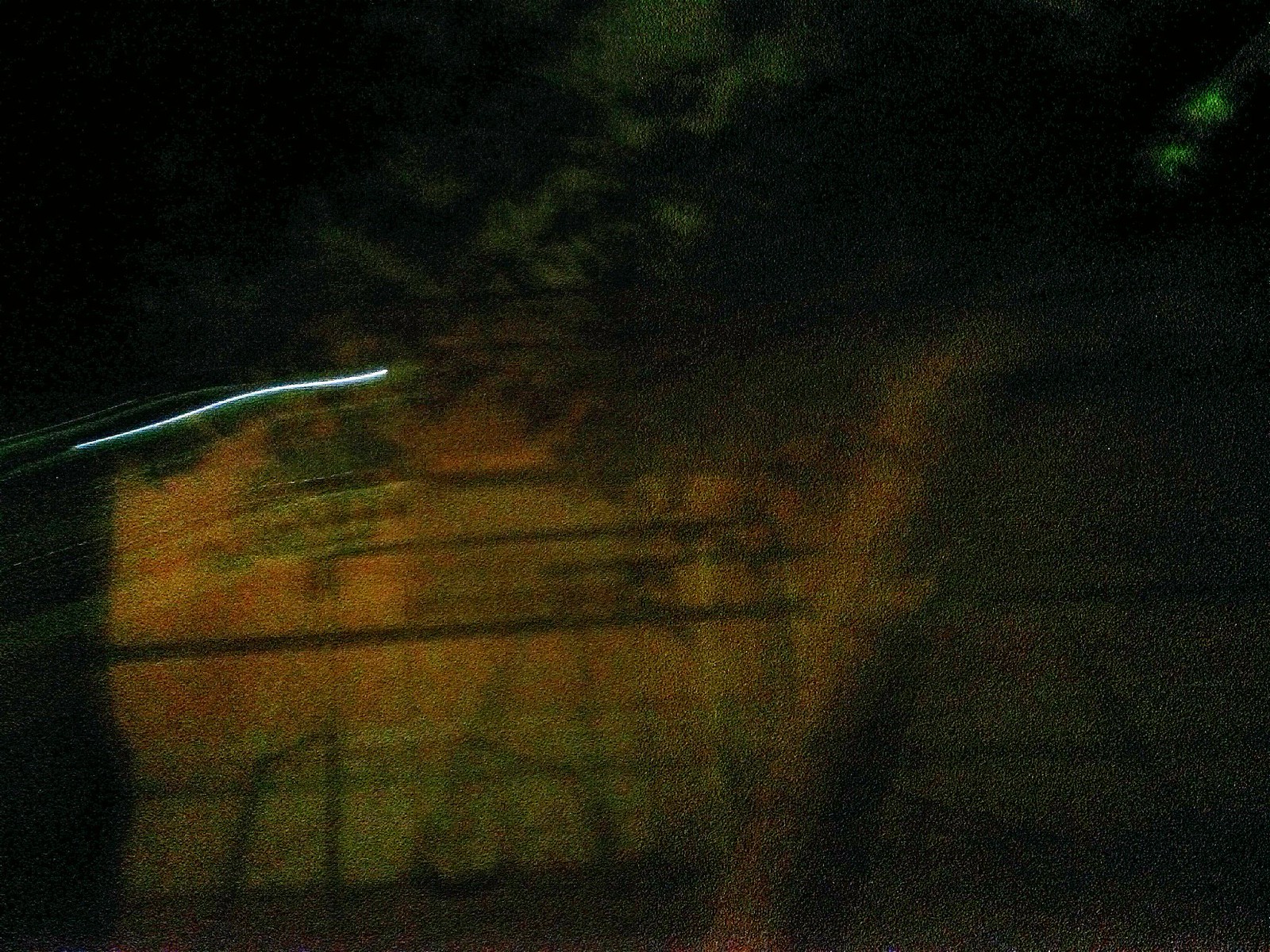The image is a grainy, blurry color photograph taken at night, with most elements indistinguishable due to motion blur. The scene appears to be an outdoor setting, dominated by a dark, almost black background interspersed with dull pastel colors. In the bottom left-hand corner, a blurred rectangular shape emerges in dark orange, red, and several shades of green. This shape is accompanied by a strikingly bright white line, likely a streak of light caused by camera movement, running horizontally across its top. 

On the right side, starting from the middle, a tree-like structure leans at a 26-degree angle to the right. Its canopy, or collection of leaves, is made up of greenish, lighter gray patches, though it's indistinct due to the graininess. In the background, partially obscured by the blur, there appears to be a swing set with a single swing hanging, framed by what looks like a chain-link fence. Above this swing set, there are two slightly brighter green dots at the top right corner of the image. Additionally, the presence of an orange-colored, nondescript large building can be inferred, though its details are unclear. The entire photograph retains an enigmatic quality, melding abstract elements with faint hints of an outdoor nighttime scene.